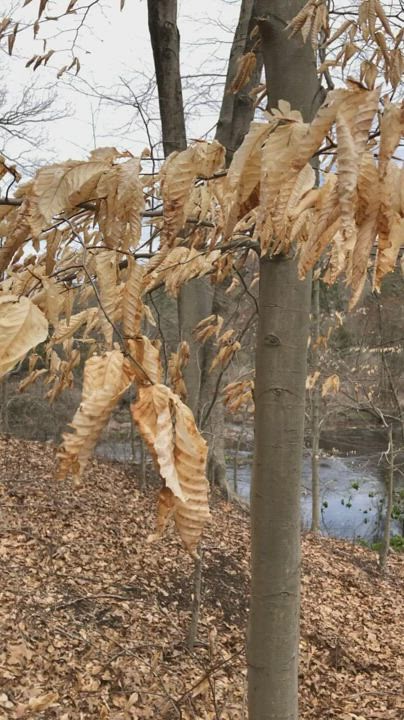This captivating photograph showcases a serene autumn landscape in what appears to be a state park, possibly in Pennsylvania. The foreground is dominated by a slender tree trunk with branches extending upwards, cloaked in yellowish-golden leaves that create a contrasting canopy against an overcast sky filled with light gray clouds. The ground beneath this tree is blanketed with a mosaic of dry leaves, broken only by occasional patches of dirt.

As your gaze moves beyond the foreground, a tranquil pond comes into view, its calm, clear water reflecting the muted fall colors. The pond is bordered by a gently sloping hillside adorned with an array of trees, some still holding onto their autumn leaves while others stand bare. Just left of center, a stone bridge spans the water, adding a rustic charm to the scene.

In the upper reaches of the photograph, wisps of branches and leaves from distant trees frame the image, accentuating the forested backdrop that stretches beyond the pond. The setting exudes a timeless, peaceful atmosphere, capturing the essence of fall with rich details and natural beauty.